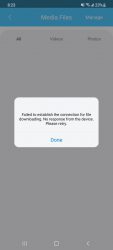This image depicts a cell phone screen with a very poor resolution, making the text and details difficult to decipher. At the top of the screen, there is a dark blue notification bar with white symbols, presumably indicating cell phone signal, Wi-Fi, and battery level, which appears to be around 31% or 32%. Below this, a bright blue band stretches across the screen, featuring a back arrow on the left and some white text in the center, although the exact wording is unclear.

The main background is gray with three black words near the top, but these words are indecipherable due to the low resolution. A white pop-up window has appeared on the screen, containing several lines of black text and a blue button at the bottom that most likely says "Done."

At the very bottom of the screen, the phone's navigation bar is visible, including three horizontal lines, a square, and a back arrow, but these are also blurred. The overall color scheme includes dark blue, bright blue, white, black, and gray. The image quality is poor, making all elements, both small and large, difficult to read.